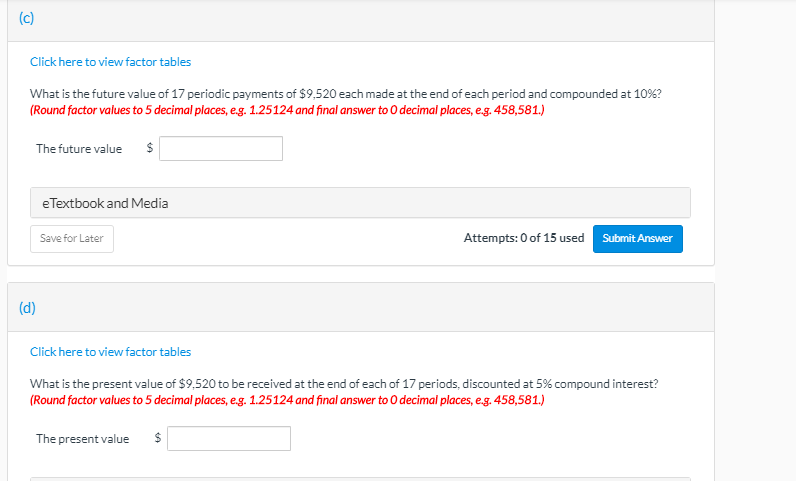This is a detailed screenshot of an online test or quiz, most likely for a high school or college-level course. The interface features a primary window with a light gray background. At the top of this window, there’s an interactive prompt labeled "Click here to view factor tables," suggesting that students may access additional resources if needed.

The first question presented in the screenshot reads: "What is the future value of 17 periodic payments of $9,520 each made at the end of each period and compounded at 10%?" Below this question, there is a designated box where students are expected to enter their answer.

Following this, the second question asks: "What is the present value of $9,520 to be received at the end of each 17 periods discounted at 5% compound interest?" Again, a text box is provided for entering the response.

Overall, the screenshot captures a segment of an evaluative assessment aimed at testing students' understanding of financial concepts related to future and present value calculations.